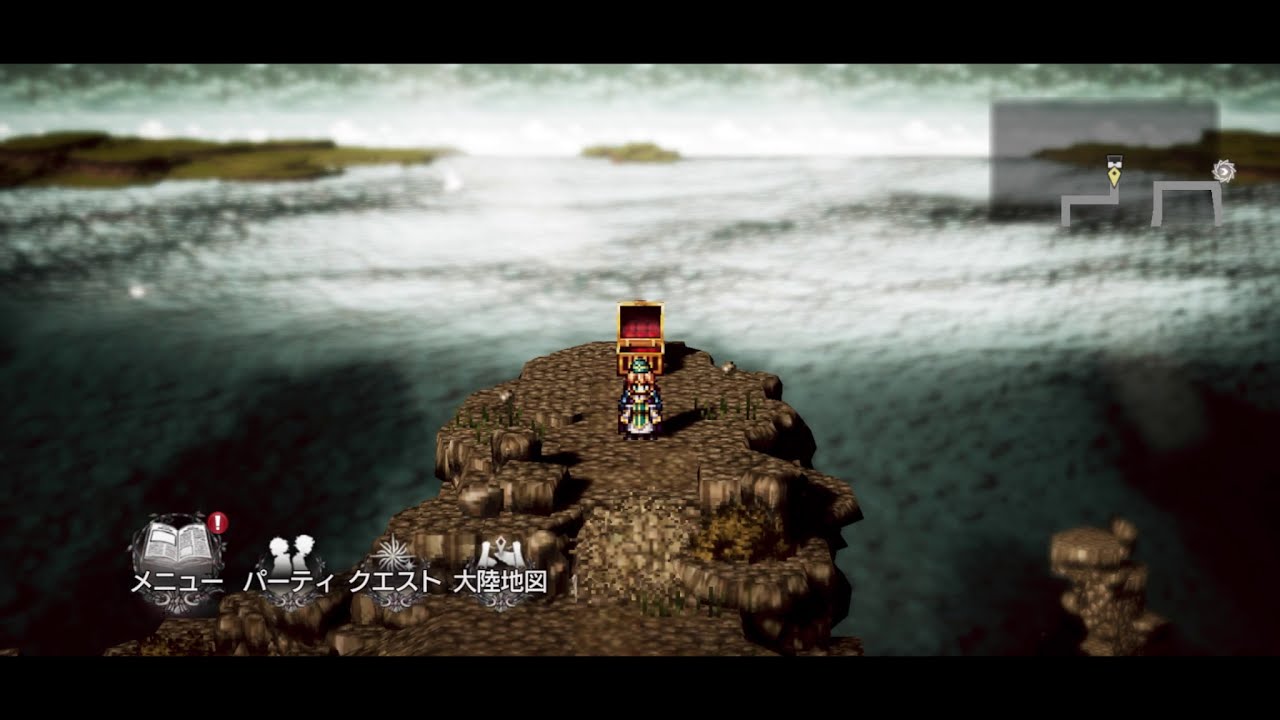In this detailed scene of a 3D adventure video game, a character resembling a princess or a maiden, identifiable by her red hair, cape, and possible tiara, stands on a rocky outcropping overlooking a gray and cloudy ocean. Positioned in front of her is an open treasure chest adorned with a golden border and a red hue. The surrounding backdrop features dramatic cliffs over a waterway, which include distinctive landmarks such as a green plateau on the left, a small island in the middle, and a large stone rectangular building or fortress on the right. The sky above is a mix of gray, blue, and white. On the bottom left of the screen, there are several icons and text written in an Asian language, possibly Japanese. These icons include a book with a red exclamation point, two figures with their backs to each other, a sunburst or firework image, and two scrolls. Additionally, a semi-transparent mini-map with navigation lines is visible in the top right corner, helping guide the player through the scenic environment.